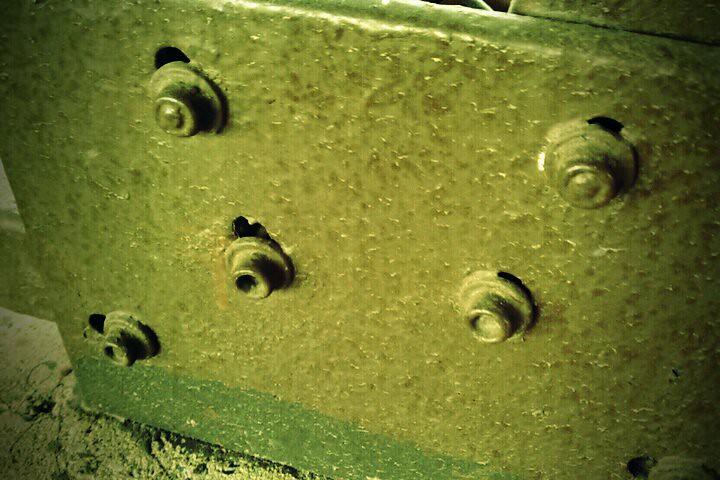The image presents a close-up view of a metallic object positioned centrally against a stone or concrete-like background, suggesting an industrial setting. The primary subject is a gray-green metal plate, occupying most of the frame. The lower portion of the plate, roughly the bottom fifth, exhibits a darker and more pronounced green hue. Affixed to this plate are five or six screws or bolts, with some gaps visible around their edges, indicating they may not be perfectly aligned or fully backed by metal. The floor beneath the plate displays a mix of gray and green tones, with patches of what appears to be dripped green paint. While the scene's function remains unclear, it is evident that the metal plate is securely fastened, possibly to a wall, with hints of the surrounding environment visible at the edges of the image.